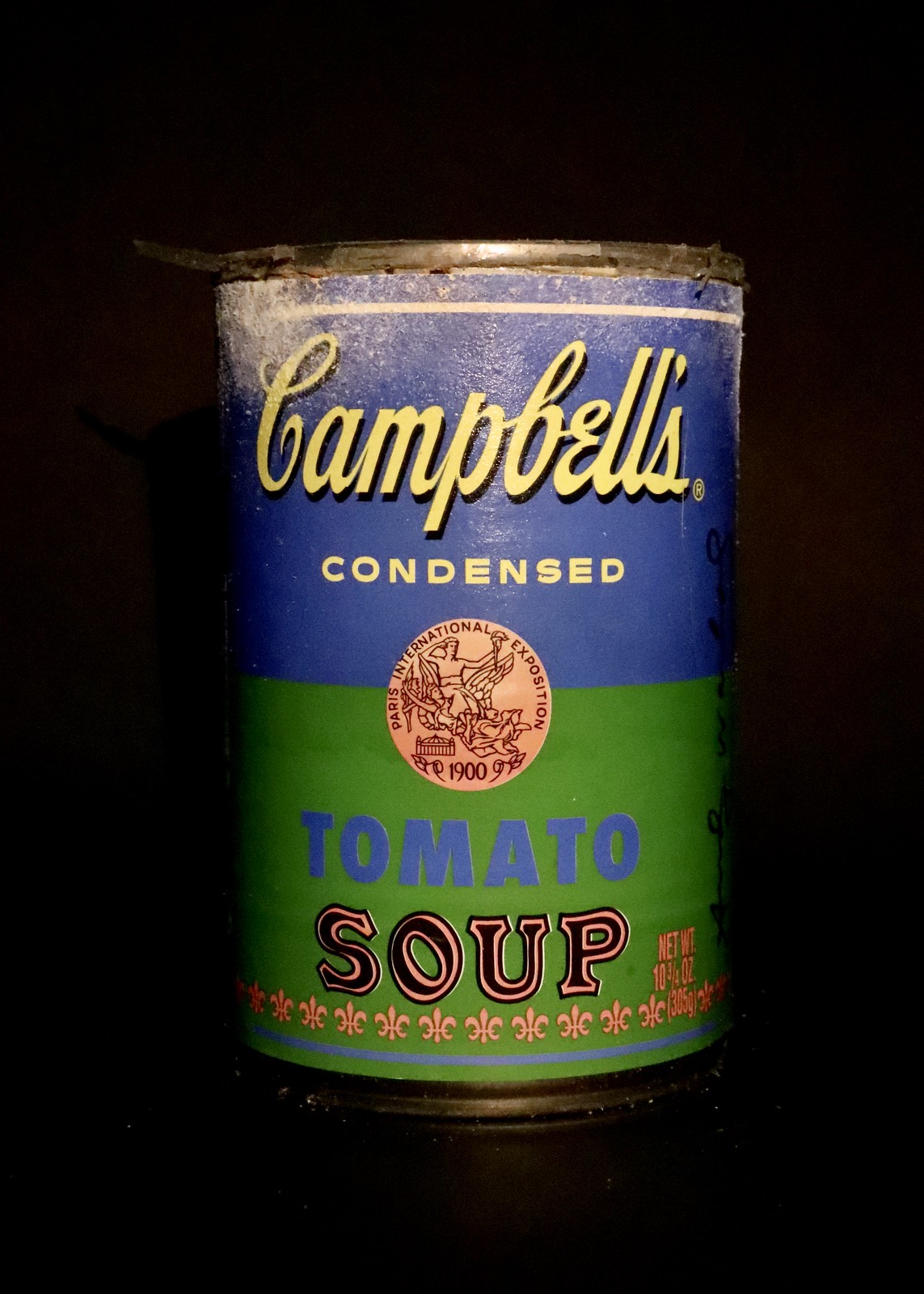The photograph features an old, possibly vintage, can of Campbell's Condensed Tomato Soup set against a stark black background. The can itself is worn, with frayed edges, and appears to be dusty, suggesting it's been stored or exposed to the elements for some time. The can is divided into two distinct halves: the top half is a faded blue color and the bottom half is light green.

At the very top of the can, "Campbell's" is written in cursive yellow lettering, while "condensed" appears below it in non-italic white letters. Separating the blue and green segments is a prominent gold circular emblem that reads "Paris International Exposition" and the year "1900," and it depicts a figure in a carriage being pulled by what appear to be angels or mythical creatures.

On the green lower half of the can, the word "tomato" is displayed in blue letters, and "soup" is printed in black with gold accents. Gold symbols resembling fleur-de-lis or possibly corn husks are arrayed near the bottom of the can, followed by a thin blue stripe that outlines the base. The label also notes the net weight as "10 and 3/4 ounces." Overall, the can's rusty and peeling condition, combined with its unusual colors, clearly signals its age and historical value.